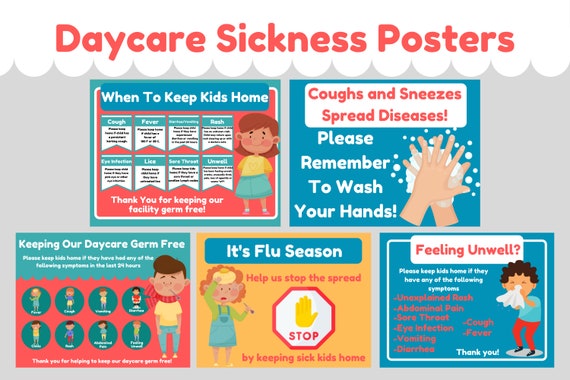The image is a detailed illustration of a set of five daycare sickness posters, prominently titled in large red font at the top, "Daycare Sickness Posters." Each poster is filled with vibrant colors ranging from dark blue to light blue, orange, and red, and they feature cartoonish illustrations that depict children, hygiene practices, and common sickness symptoms.

The five posters are arranged in a grid from the top left to the bottom right:

1. **When to Keep Kids Home**: This poster lists symptoms such as cough, fever, rash, eye infection, lice, sore throat, vomiting, diarrhea, and general unwellness as indicators for keeping children home from daycare.
2. **Coughs and Sneezes Spread Diseases**: Illustrated with someone washing hands, it emphasizes the importance of hand hygiene to prevent the spread of illnesses.
3. **Keeping Our Daycare Germ-Free**: Aimed at daycare employees and parents, it asks to keep children home if they have had fever, cough, vomiting, diarrhea, chills, rash, abdominal pain, or feeling unwell in the last 24 hours.
4. **It's Flu Season**: This poster highlights measures to stop the spread of flu by keeping sick children at home.
5. **Feeling Unwell**: Similar to the first poster, it advises keeping kids home if they exhibit symptoms like unexplained rash, abdominal pain, sore throat, eye infection, vomiting, diarrhea, cough, or fever. 

These posters collectively serve as a comprehensive guide for maintaining a healthy daycare environment by outlining clear guidelines for parents and staff.